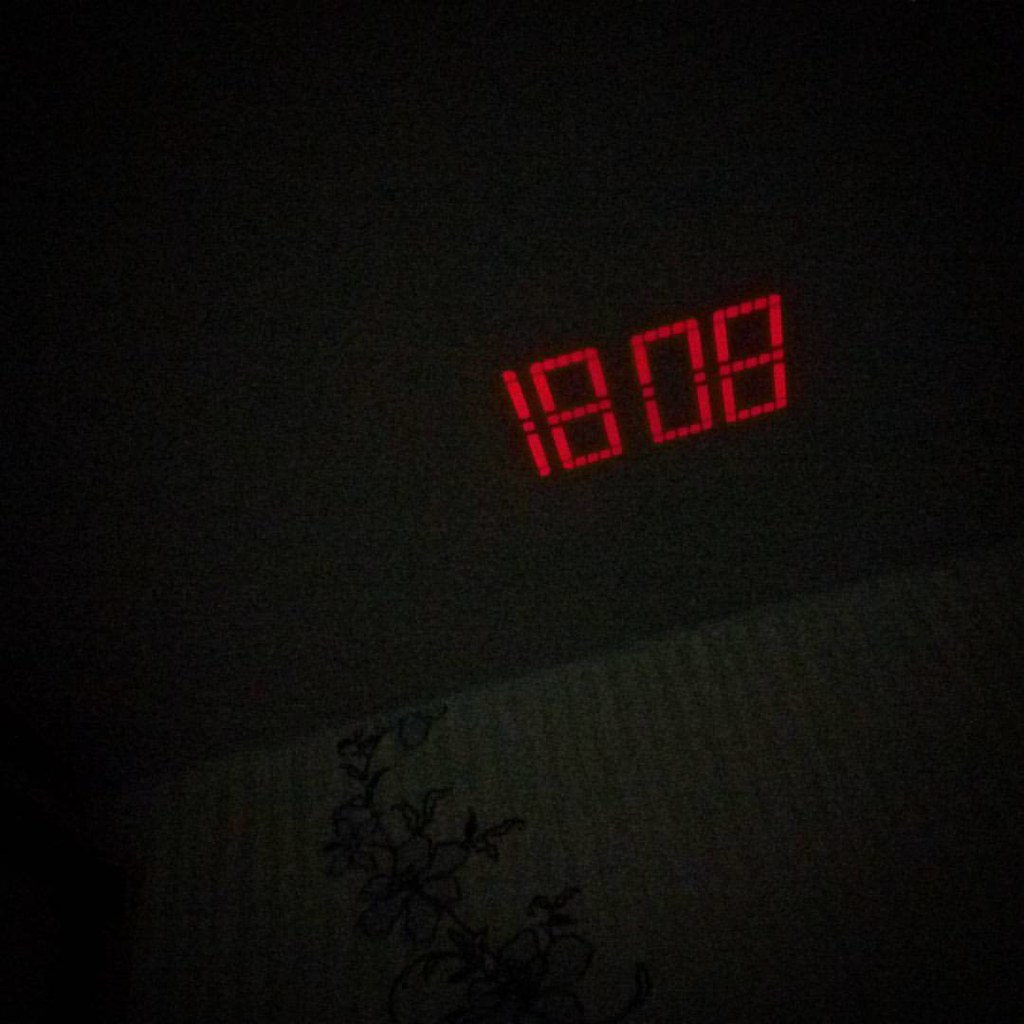This image captures an upward, angled view of a digital clock projection on a ceiling at night. The large, red digital numbers displaying "18:08" are projected slightly off-center to the right, angled downwards towards the left. The ceiling, colored in a dark or tan shade, contrasts with the vivid red numerals. The photo's low lighting suggests it was taken in a dimly-lit or nighttime setting. The bottom portion of the image reveals a pinstripe-patterned wall, with a white or tan base color accented by darker tan or green stripes. A black and gray flower motif adorns the wall, curving gracefully from the bottom center up towards the right, concluding near the ceiling.